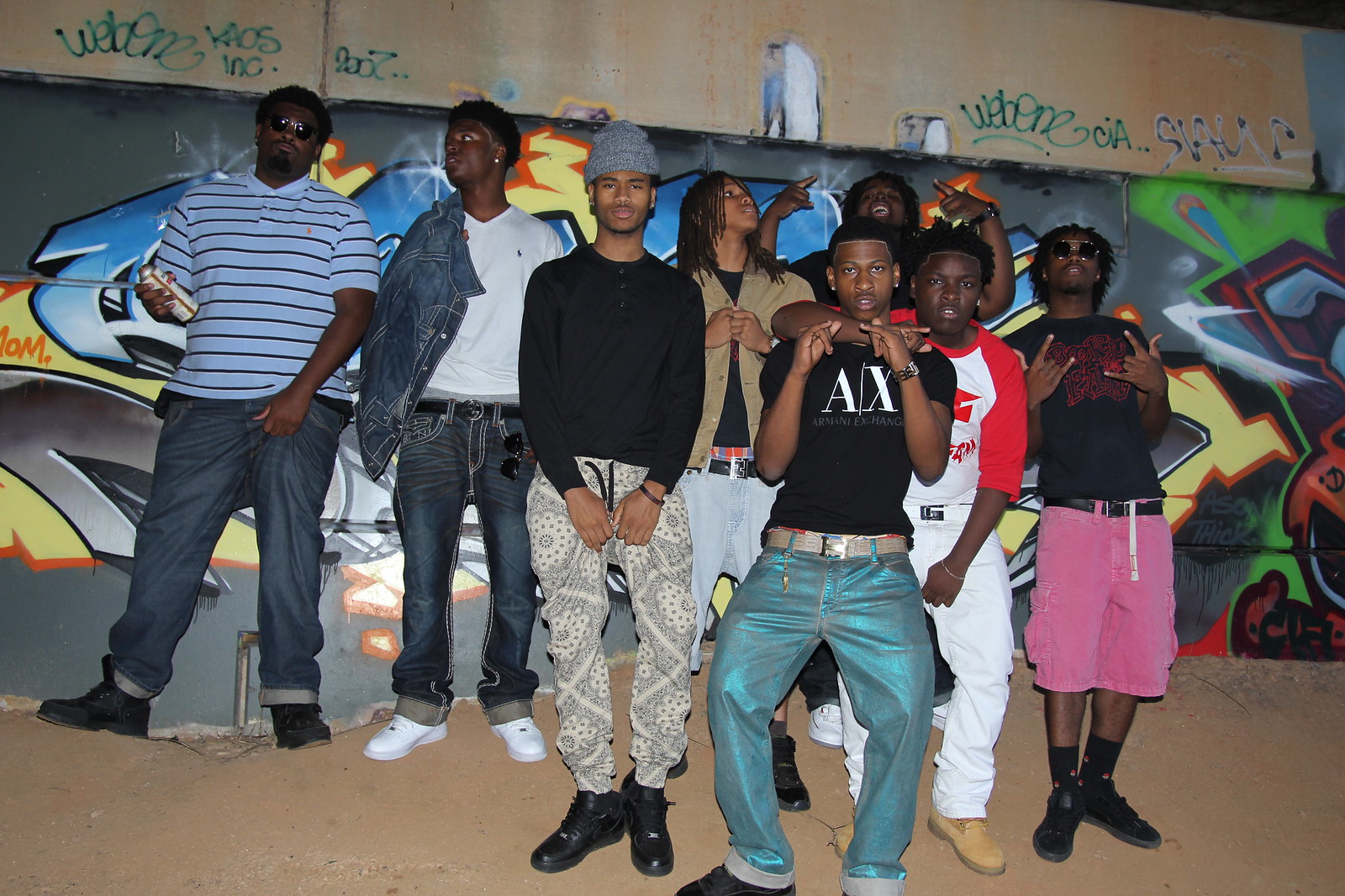The image depicts eight young African-American men standing in front of a wall covered with colorful and intricate graffiti. The vibrant background features an array of blues, greens, reds, and some less orderly tags at the top. The men are casually dressed and appear to be enjoying themselves, almost as if they're posing for a group photo, potentially even for a music video.

Starting from the left, the first man is wearing sunglasses, a blue striped collared shirt, blue jeans, and black sneakers. Next to him is a man in a denim jacket over a white shirt, with matching blue jeans and white sneakers. The third man is sporting a grey hat, a black long-sleeve shirt, and grey-white paisley pants with black sneakers. Following him is a man with long braids, donning a tan shirt and blue jeans.

Behind this main row, slightly in the background, is another man whose head is visible as he raises his arms, appearing to greet the camera. In the forefront, a gentleman wears an Armani Exchange black shirt, shiny blue-green pants, and black sneakers. To his right, another man dressed in a white and red shirt paired with white pants and work boots catches the eye. Finally, on the far right, a man with small plaits in his hair, sunglasses, a black shirt with a red design, pink shorts, black socks, and black sneakers holds up a "devil horns" hand gesture, contributing to the laid-back and cheerful vibe of the group.